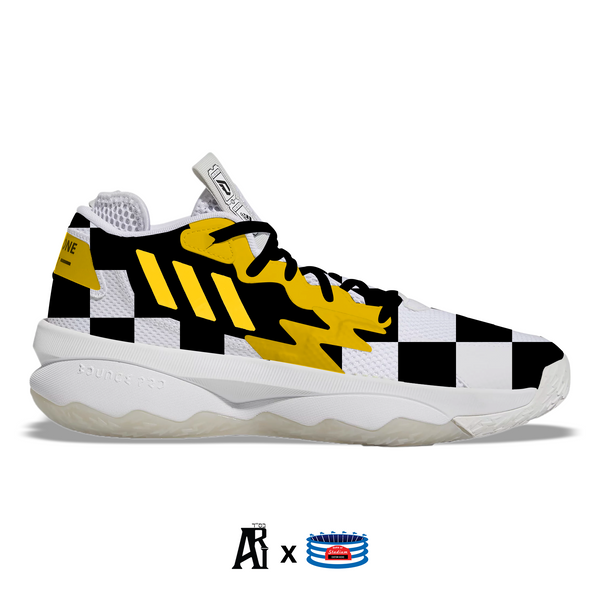This full-color image showcases a tennis shoe, primarily black and white in color with a checkered pattern adorning the main body. The shoe, featuring a thick white rubber sole, faces to the right. Adding a vibrant touch, the sides of the shoe incorporate yellow accents, alongside black Adidas-style diagonal stripes set against a black background. The black laces contrast with the shoe's design, and the tongue prominently sticks up, revealing a hint of mesh at the back.

The image is devoid of a definitive shape, border, or background, set against the plain whiteness of the screen. At the bottom, additional digital elements include a capital 'A', 'R', and an 'X' in black. Also present is a circular stadium-like logo with blue flags at the top, darker blue interior, concentric blue and white rings, and a small red emblem. The shoe’s shadow is visible on the surface, adding depth to the otherwise stark composition.